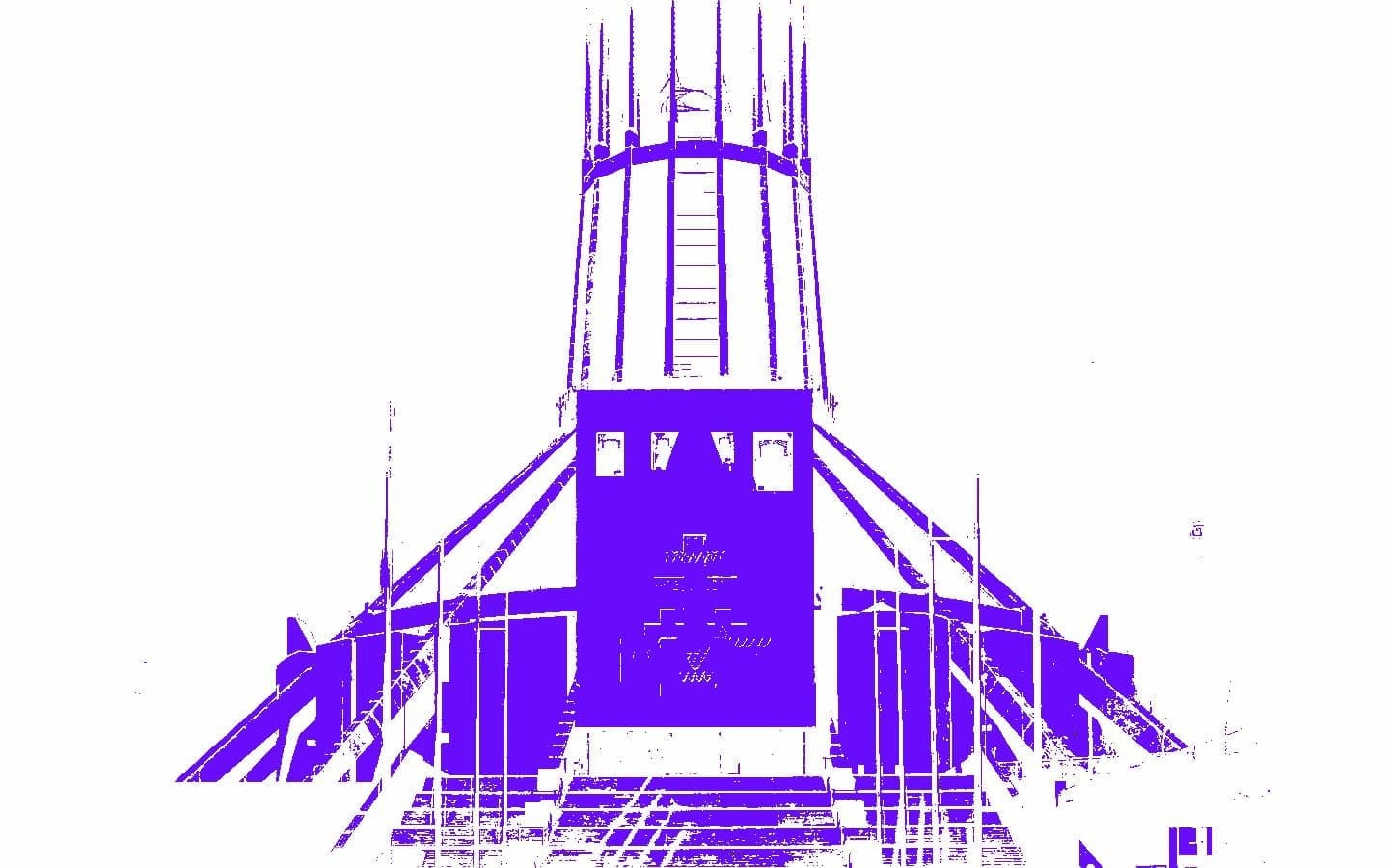The image features a monochromatic purple structure set against a stark white background, emphasizing the total lack of borders. Dominating the bottom of the scene is a staircase that leads up to a series of doors, suggesting an entryway to a mysterious building. At the center above the stairs sits a large purple rectangle accented with unidentifiable white markings. Above this rectangle, a tall, cylindrical tower extends upward, adorned with what could be interpreted as a ladder or metal bars encircling it. Flanking the tower are two angled support beams, reinforcing its imposing presence. The scene's sparse yet intricate elements, including poles that might support lighting, contribute to an otherworldly architectural assembly, rendered surreal by possible digital effects and an inverted color scheme.